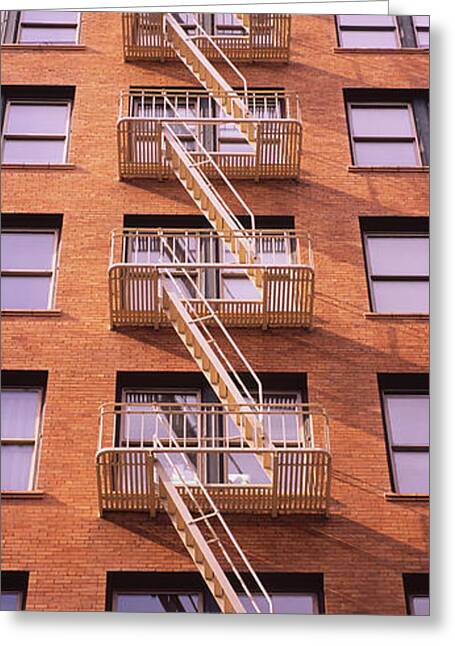We're looking at the side of a multi-story, red brick building with numerous double-paned windows. The building, possibly extending beyond the photo's edges, displays five floors, though there are indications of more above and below due to visible ladder bases. Centered in the façade are four metal wire balconies, all equipped with yellow fire escapes. The windows are recessed with gray trim, mostly dark with one exception where a light is visible inside. The fire escapes and balconies are prominently painted a cream or light buff color, adding a distinct contrast to the building's deep amber brickwork.